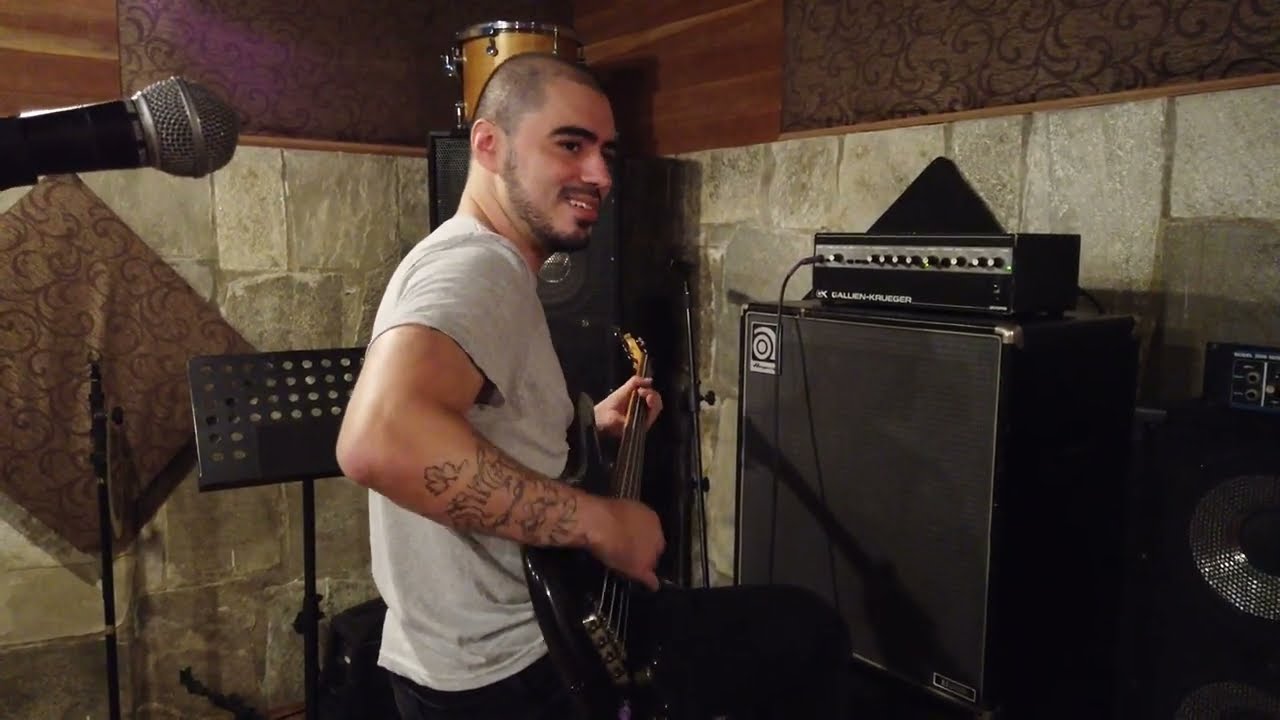The image depicts a white man with short hair, a goatee, and a hint of facial hair, dressed in a light gray t-shirt and black pants, playing a black guitar in what appears to be a basement or potentially an unfinished garage. The environment suggests a makeshift recording studio, with stone walls, visible insulation, and wooden ceiling components. The man, seen from a side profile as he looks to his right, has tattoos on his right forearm. He is seated, resting the guitar on his left leg while strumming the strings with his right hand, presumably using a pick. Surrounding him are various pieces of musical equipment, including a large black speaker on the right, an amplifier with a plug above it, and a music stand. On the left, a microphone is jutting out, although it is not being used. The room is filled with an assortment of recording paraphernalia, emphasizing the creative and informal setting.